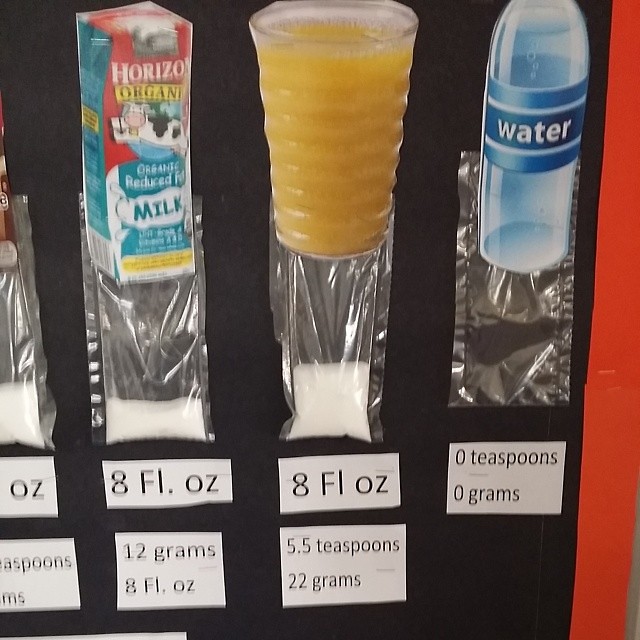This image is a photograph resembling a school science project that visually demonstrates the sugar content in various beverages. The display features a black background with a red border, possibly made from stapled paper, giving it a textured look. The board is organized with real images of different drinks, each accompanied by a small plastic baggie containing a proportional amount of sugar. 

On the far right, there's a bottle of water with an empty baggie underneath it, labeled "0 teaspoons, 0 grams of sugar." To its left, a glass of orange juice is depicted, with the corresponding baggie filled about one-third of the way and labeled "8 fl oz, 5.5 teaspoons, 22 grams of sugar." Next, a bottle of Horizon organic reduced fat milk is shown, its baggie filled about one-fifth full, marked "8 fl oz, 12 grams of sugar." On the far left, partially out of frame, there's evidence of another beverage, possibly chocolate milk, but the details are unclear. Each baggie is either stapled or glued to the board directly below the respective drink image.